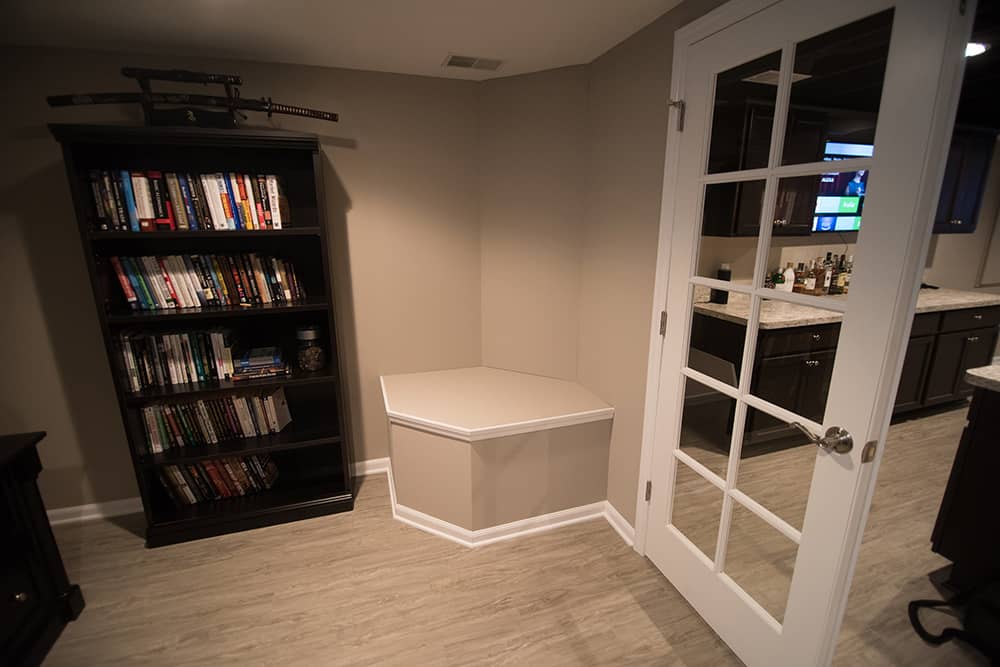This image depicts a well-lit basement room with beige-tan walls and light beige or light gray wood flooring. Central to the room is a dark wood bookcase filled with brightly colored books, adding a vibrant touch to the space. Adjacent to the bookcase is a seating area without cushions, indicating a casual, unfinished hangout spot, possibly a man cave. A prominent feature of the room is the clear glass door with multiple panes and a wood frame, which opens into another room. This adjoining area appears to be a kitchenette or bar, equipped with cabinets and a TV, contributing to the room's relaxed, recreational atmosphere. Overall, this image showcases a cozy, multi-functional basement area designed for leisure and socializing.